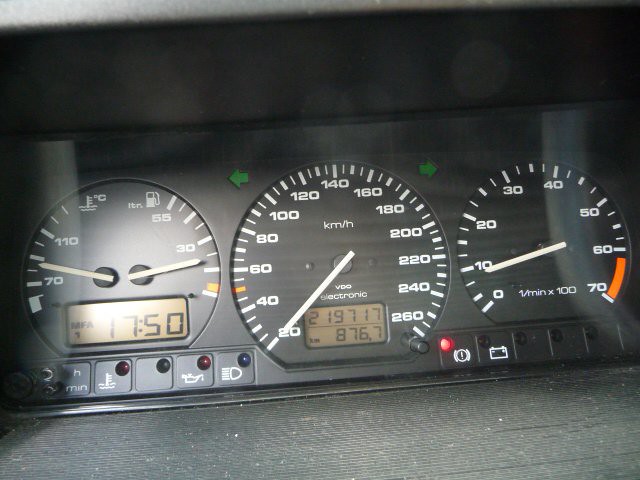This horizontal close-up image captures three circular gauges on an automobile dashboard. The top and lower edges of the dashboard are gray, with the gauges set into a black frame recessed within a leather-textured plastic surface. From left to right, the gauges are:

1. A combination temperature and fuel gauge. The digital readout on this gauge displays "MPA," which reads 1750. Below the gauge are five buttons with indicator lights showing various minimum temperatures. One button features a red light with a temperature gauge symbol. Another button features an oil can icon with an oil indicator light in the upper right corner. There is also a green light indicator for possible parking lights.

2. The center gauge is the speedometer, marked in kilometers per hour. At the top corners of this gauge are green turn signal arrows for left and right indications. Below the speedometer is a digital readout, including the odometer displaying 219,717 kilometers and an auxiliary trip meter reading 876.7 kilometers.

3. The right gauge is a tachometer with a red light indicator at the bottom right, possibly related to the steering system. There is also a small button-like battery indicator with a light in the upper left corner.

All three gauges have black faces with white letters and numerical markings. The temperature gauge is shown in degrees Celsius and the fuel gauge ranges from 55 down to below 30. Both the temperature and fuel gauges use needle indicators for measurements.